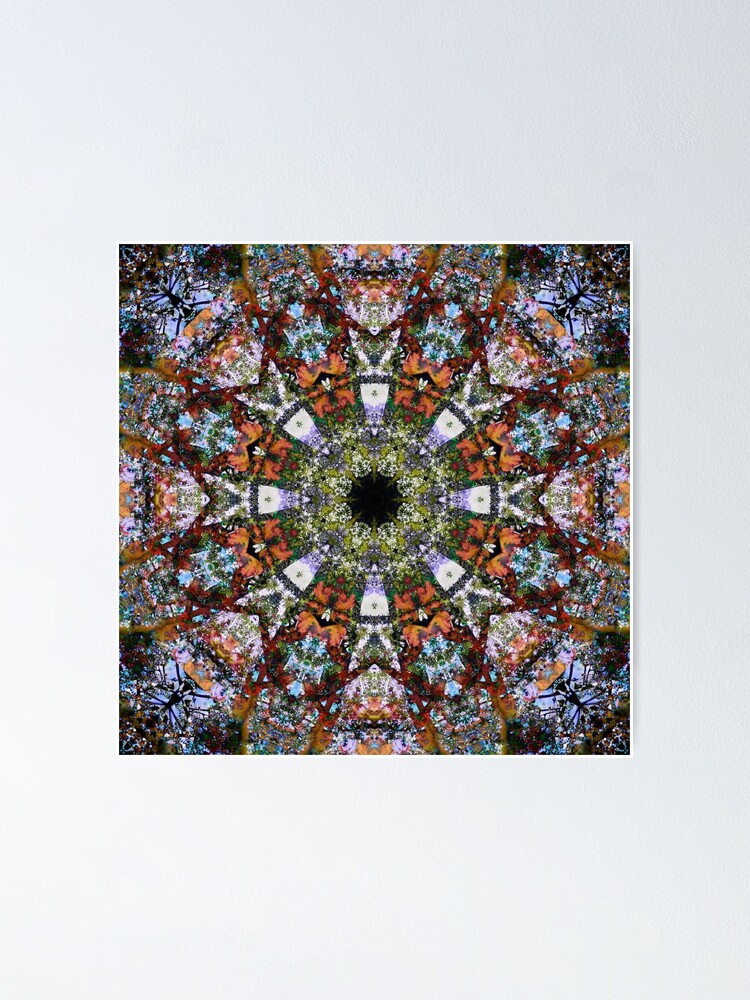The image appears to be a complex, symmetrical kaleidoscope view featuring geometric patterns and vibrant colors. At the center, there is a dark black circle, encircled by a green ring and a purple ring, followed by an area of orange rectangles. These elements replicate outward in an eightfold symmetrical pattern, creating a repetitive design that includes bands of dark red, lighter orange, and black hues, suggesting a continual spreading effect. Additionally, eight golden rods radiate from the black center towards the edges of the image. In each corner—top left, top right, bottom right, and bottom left—there is a lavender-tinted dragonfly silhouette, adding a distinctive touch to the intricate, floral-like arrangement. The entire image exudes femininity and intricacy, evoking the nostalgic experience of looking through a child's toy kaleidoscope, where the geometric patterns and vibrant colors shift and repeat, creating mesmerizing designs.